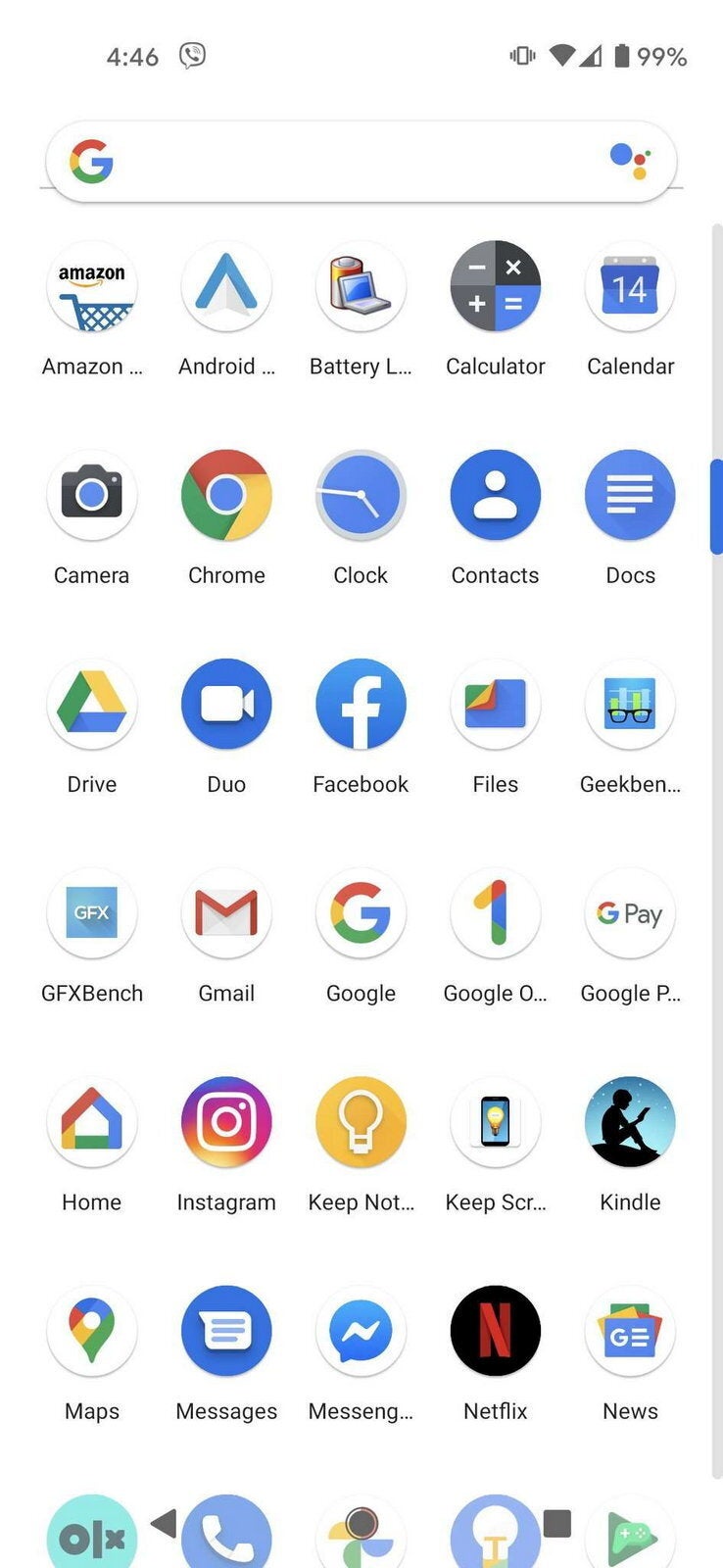A screenshot from a phone captured at 4:46 AM with a battery level of 99% is shown in the upper left-hand corner. Below this, a search bar featuring the Google "G" icon on the left end is prominently displayed. The main section of the image showcases a home screen filled with numerous app icons arranged in a grid. Beginning from the top left corner, the icons include: Amazon, Android, Battery, Calculator, Calendar, Camera, Chrome, Clock, Contacts, Docs, Drive, Duo, Facebook, Files, Geek (name truncated with three dots), GFXBench, Gmail, Google, Google One, Google Pay, Home, Instagram, Keep, Notes, Keep Screen, Kindle, Maps, Messages, Messenger, Netflix, and News. Additionally, there is another row of five app icons at the bottom, but only the tops of the corresponding symbols are visible, leaving the app names cut off and unclear.